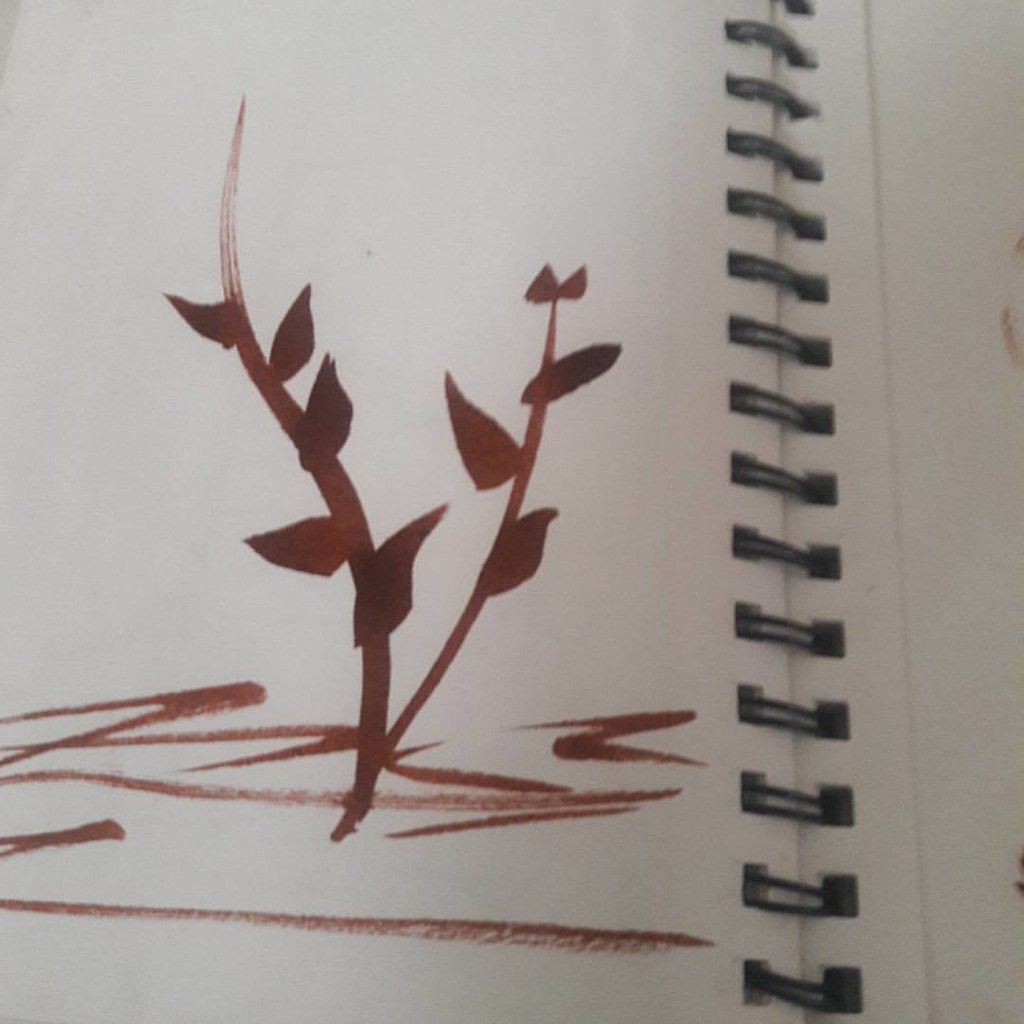This is a color photograph of a high-quality sketchbook or binder featuring an artistic drawing. The sketchbook is open, revealing its unique black, multi-ring metal binding that uses square holes, with approximately 30 rings visible. The image captures primarily the left page, showcasing a simple yet detailed artwork in dark maroon ink or paint, which could be marker or watercolor. The drawing consists of two plant stems, possibly thyme branches, emerging from a hastily scribbled ground. The stem on the left has five leaves, while the stem on the right has three leaves with two smaller leaves clustered at the top. The paper appears to be high-quality, suitable for various forms of artistic expression. The right-hand page is mostly out of the frame, but a small, dark maroon line is visible, suggesting another part of an artwork. A faint tear line is noticeable along the edge, indicating where a previous page may have been removed.